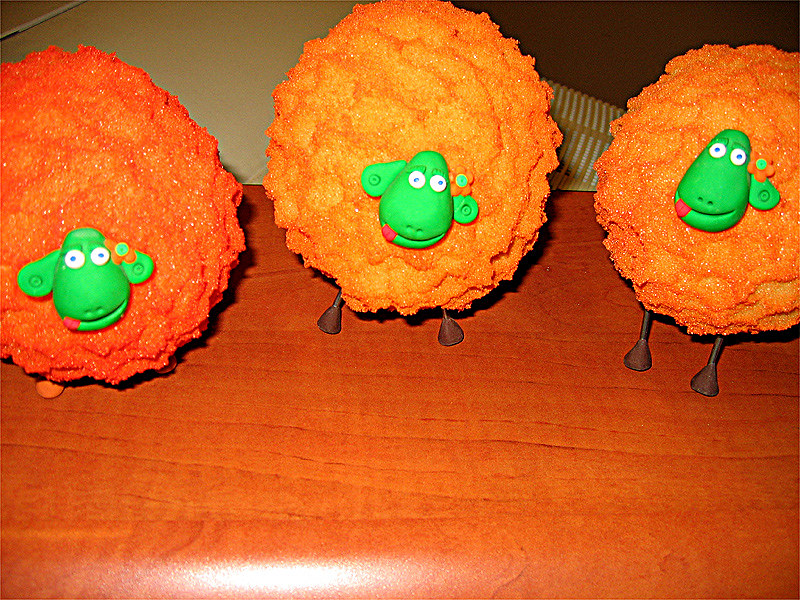In this photo, a cream-colored background contrasts with a shiny, brownish-reddish wooden surface in the foreground, possibly a kitchen table. Atop this surface sit three whimsical, handcrafted sheep figurines. The bodies of these sheep are vividly orange, reminiscent of oversized Cheetos cheese puffballs or chunks of cake coated with fluffy orange frosting to simulate thick fur. Each sheep possesses a green face with large eyes, prominent ears, and a tongue hanging out of its mouth. Additionally, each has an orange flower adorning its left ear. The sheep stand upright on small, brown legs, which look almost like golf pins, adding a playful touch to the overall scene.